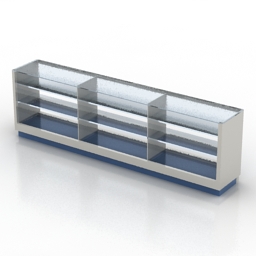Set against a minimalistic background with a white upper half and a light gray lower half, the image depicts a long, narrow shelving unit or display case. Positioned at an angle from the top left to the bottom right, the unit features three sections separated by gray partitions, each containing glass shelves. Constructed with a silver metal frame, the bottom of the shelving unit and its stand are dark blue. The image also shows some reflection of the unit on the floor, adding to the clarity and simplicity of the scene.